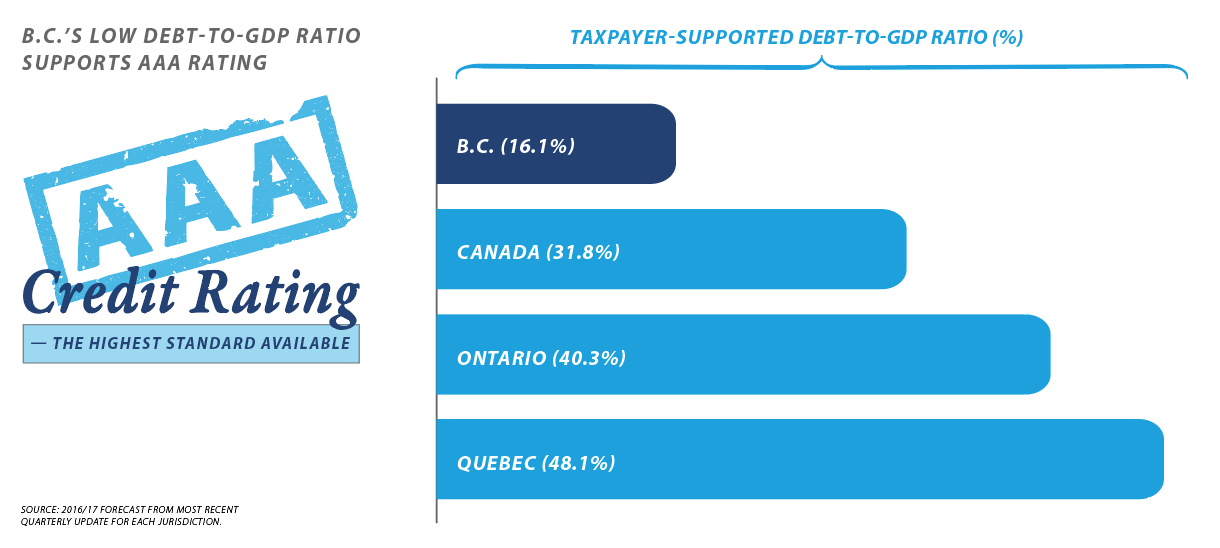This infographic illustrates the taxpayer-supported debt-to-GDP ratio percentages across various jurisdictions. Highlighting British Columbia's (BC) fiscal responsibility, the text on the left states, "BC's low debt-to-GDP ratio supports AAA rating," complemented by a stamp indicating "AAA credit rating, the highest standard available." The bar graph details BC's comparatively low debt-to-GDP ratio at 16.1% (depicted in dark blue), significantly lower than Canada at 31.8%, Ontario at 40.3%, and Quebec at 48.1% (all depicted in light blue with white text). The source at the bottom left references the 2016 to 2017 forecast from the most recent quarterly update for each jurisdiction.